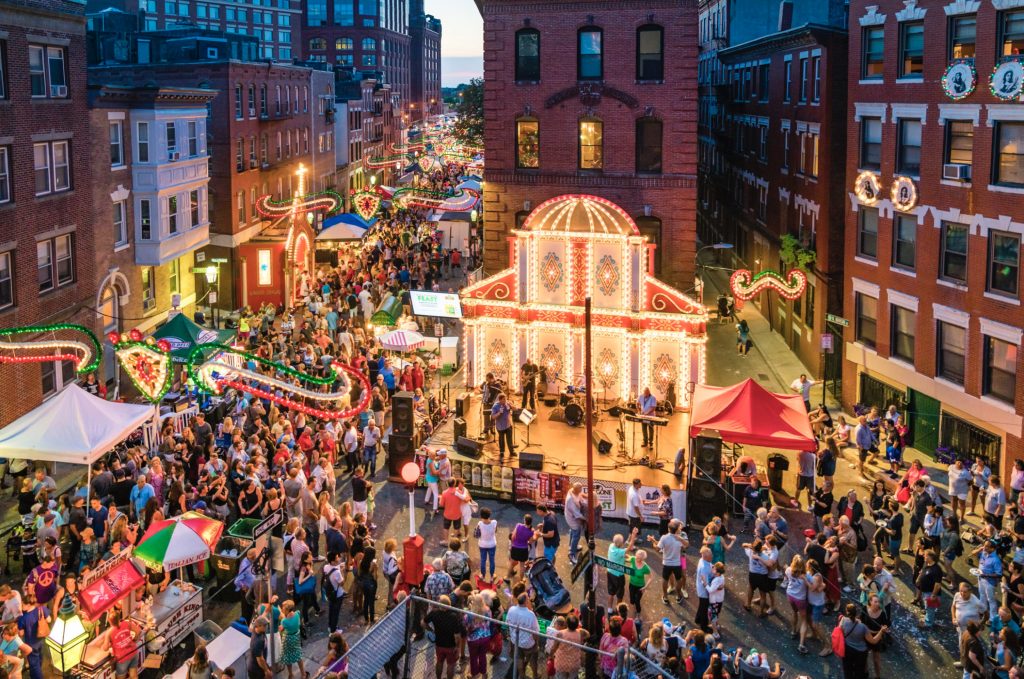The vibrant image captures a bustling street festival from a top-down perspective, likely taken from the fourth floor of a nearby building. The scene centers around a stage where a band of four musicians is performing, adorned with red and gold decorations. Hundreds of people fill the square, either dancing, socializing, or simply enjoying the music. The festive atmosphere is amplified by an array of lights illuminating the area, alongside numerous stalls and tents. The street stretches into the distance, flanked by tall, brown brick apartment buildings on both sides and behind the stage. The scene is lively and colorful, suggesting a celebration or concert deep within a city's downtown area.